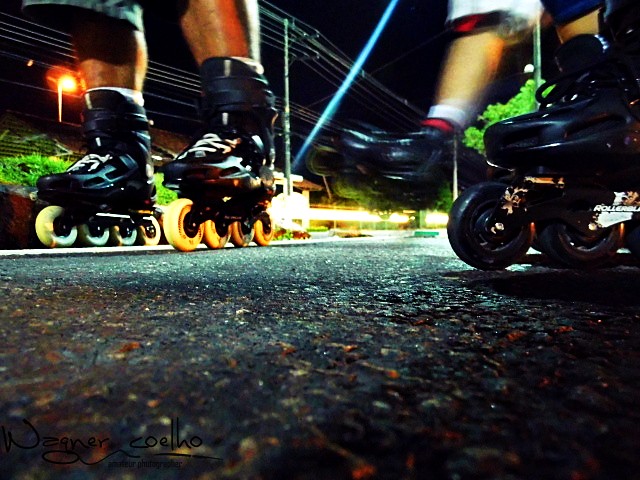This nighttime photograph, captured by Wagner Coelho, features the legs of roller skaters in motion, showcasing a vibrant scene illuminated by street lamps. The ground-level shot emphasizes the dark grey pavement scattered with fallen leaves. On the left side, a pair of roller skates with yellow wheels is worn by an adult male, while to the right, another skater is seen in black roller skates with black wheels. Above, electric poles and wires crisscross the dark sky, adding urban texture to the scene. The photographer's signature, "Wagner Coelho," and the title "Amateur Photographer" are visible at the bottom left of the image.